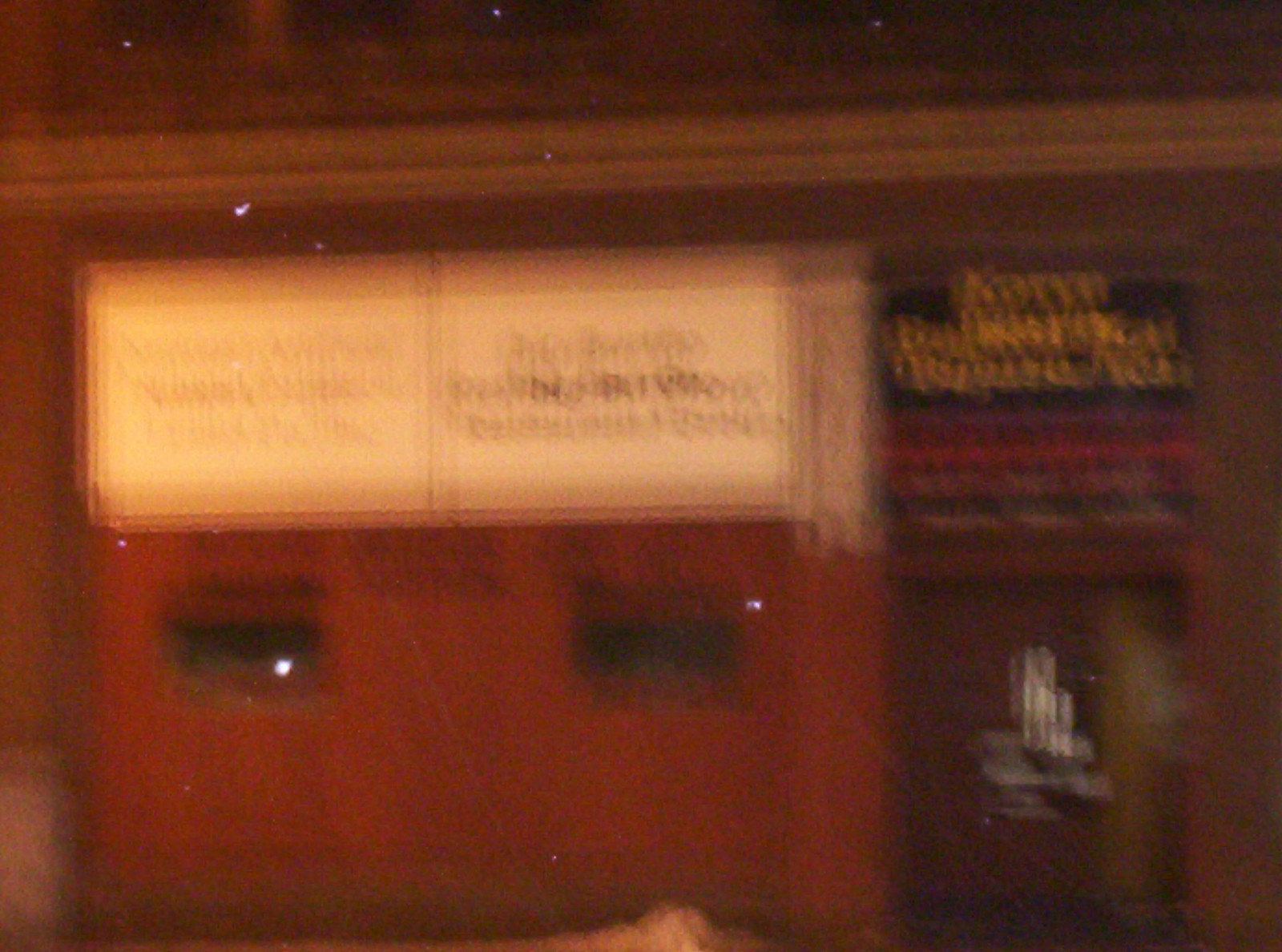This is a very blurry image of the front facade of a two-story building. The ground floor features a wide, red garage door or entrance, flanked by two windows, one on each side. Above the door, a large, rectangular white sign with a black vertical line down the center and black writing on either side is prominently displayed. To the right of this setup, there is a black sign with yellow text at the top and what appears to be red and purple writing near the bottom. Below this black sign, a glass door is visible. The top section of the photo reveals a partial view of the building's second floor, with a row of windows lining this upper level.